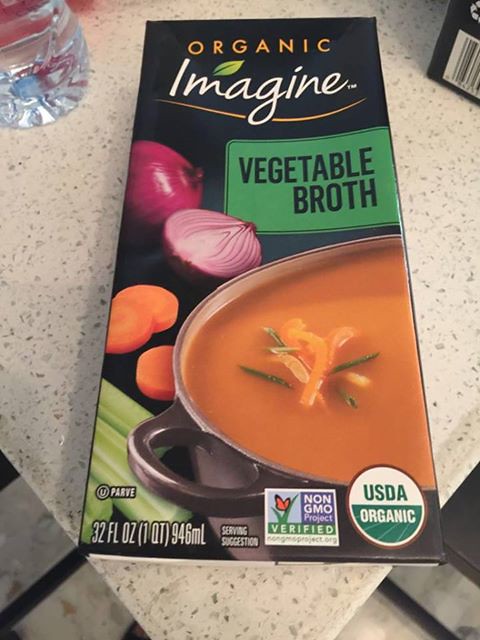This close-up image showcases a product container with a black background. Prominently displayed at the top, the word "Organic" is written in bold orange letters. Directly beneath, "Imagine" is inscribed in white lettering, highlighted by a green leaf positioned over the 'M' and an orange underline beneath the word.

The container features an array of vegetables: on the left, a whole purple onion catches the eye, followed by neatly sliced orange carrots below. Further down are several green celery sticks. Toward the right side, there's a green rectangle with the text "Vegetable Broth" written in black. Below this, a black pot filled with orange soup is depicted, with visible shreds of orange and green, likely representing the carrots and celery.

At the bottom of the container, certifications and measurements are listed: a "USDA Organic" seal, a "Non-GMO Verified" label, and volume indicators stating "32 Fluid Ounces," "One Quart," and "946 Milliliters."